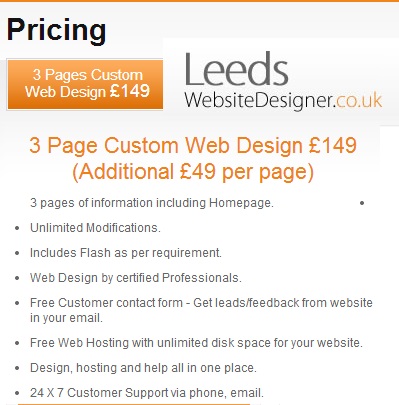The image displays an advertisement for LeedsWebsiteDesigner.co.uk with a clean white background. At the top, there is a thin horizontal orange stripe, followed by the bold black text "Pricing." An orange rectangular icon nearby advertises "Three Pages Custom Web Design £149," with additional pages offered at £49 each. To the right of this icon, the company name, Leeds, and the website URL (LeedsWebsiteDesigner.co.uk) are prominently displayed. Below, the same pricing details are reiterated, followed by a detailed bullet list in black text describing the services: 

- **Unlimited modifications** 
- **Includes Flash as per requirement**
- **Web design by certified professionals**
- **Free customer contact form**
- **Receive Leeds feedback from the website directly to your email**
- **Free web hosting with unlimited disk space for your website** 
- **Design, hosting, and help all in one place**
- **24/7 customer support via phone and email**

The heading is in orange letters, while the main text is in black, providing a clear and visually appealing contrast.